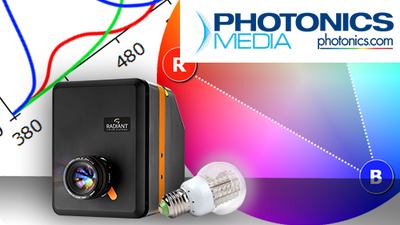The image prominently features the text "Photonics Media" in navy blue, with "Media" in all capital letters and rendered in a turquoise font. Beneath this title, "photonics.com" is also displayed. The numbers "380" and "480" are in black text, indicating specific values or measurements. The image includes several wave-like lines—blue, red, and green. Both the blue and red lines have a bell-shaped curve, while the green line trends upwards differently. Additionally, there is a white light bulb graphic and a black rectangle incorporated into the design.